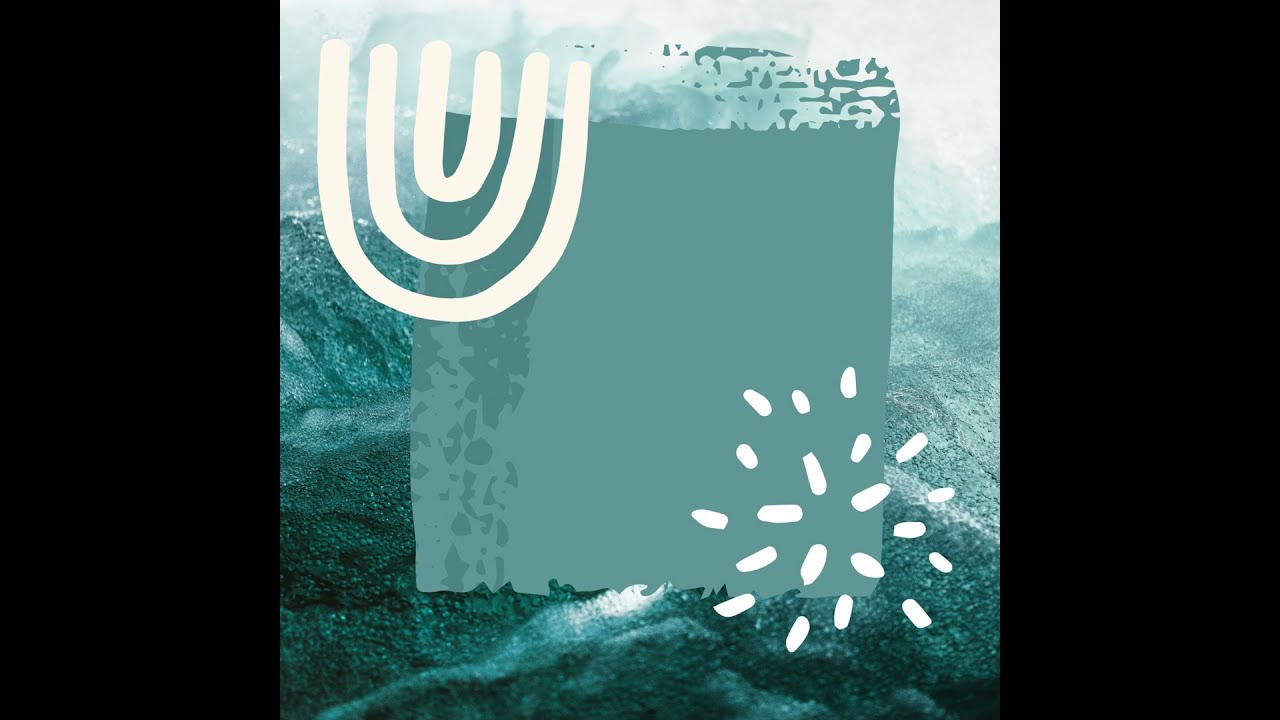The image depicts an animated design centered within a black border. Dominating the composition is a large, blue square with several white, curved scribble marks, some forming a repeated 'U' shape in the upper left corner, resembling a white rainbow with three arcs. In the lower right corner, there is a white starburst pattern of dashes. The background features what appears to be sand or a grainy rock texture with a blue tint, adding a shimmering effect. The entire scene evokes a sense of waves and movement, combining elements of blue, black, and white in a meticulously layered design.